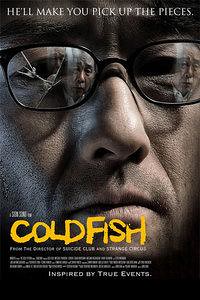The image is a detailed movie poster with a stark, black background. Dominating the center is an enlarged, close-up of an Asian man's face, emphasizing his pores and serious expression. He's wearing spectacles, with a significant detail: the left lens is cracked, revealing fine cracks, while the right lens is undamaged. Reflected in the left lens is the face of an older Asian man, adding an intriguing layer of depth to the visual composition. Above the man's forehead, a caption in white text reads, "He'll make you pick up the pieces." Centrally below the man's serious gaze, the movie title "Cold Fish" is prominently featured in bold yellow letters. Additional, less clear white text surrounds the title, hinting at themes of "suicide," "clue," and "strange circles." Beneath this text, in slightly larger white letters, is the phrase "Inspired by true events." The overall composition is framed by the black background, which extends slightly upwards on the left and right sides, creating a subtle border.